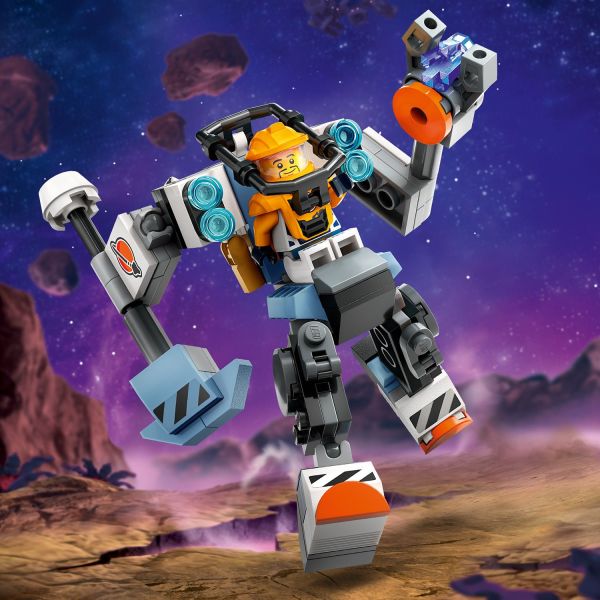The image depicts a highly detailed Lego creation set in an apocalyptic, space-themed environment. Central to the scene is a mechanical suit made entirely of Lego pieces, which houses a Lego man piloting the suit. The Lego man is attired in an orange hard hat and is securely strapped into the mech with a black pipe. The mech, which features an armored orange exterior with black and white accents, is equipped with two articulating arms. The right arm ends in versatile grabbing tools, while the left culminates in a solid, square-shaped attachment that could be a weapon or tool. The mech's shoulders are adorned with blue lights, enhancing its futuristic appearance.

Its legs, built from thick Lego blocks, are designed to articulate, giving the impression that the mech is running. The feet are composed of solid square blocks, contributing to its sturdy construction. The scene transitions into a vivid background, depicting an apocalyptic desert under a purple and pink night sky, scattered with asteroids and illuminated by meteors. The ground suggests a hostile environment with steam and gases rising from crevasses emitting purple light. The entire composition highlights the creativity and intricate detailing characteristic of Lego designs, making it worthy of a promotional image for a Lego product.